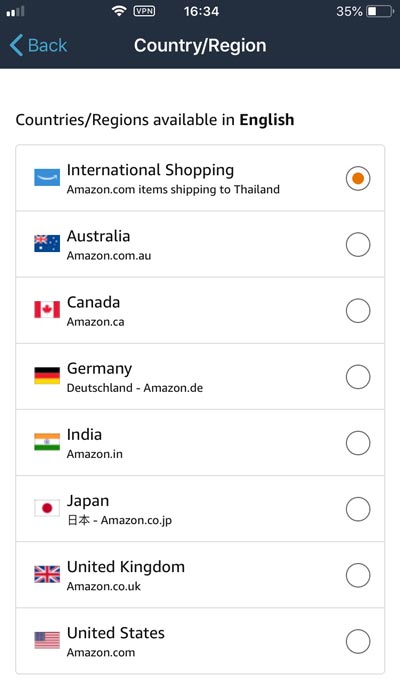A cell phone screenshot displays a settings page with various regions and options. At the top of the screen, a black horizontal bar houses several white icons typical of a smartphone's status bar. Just beneath this, there's a navigation bar with a blue left-pointing arrow resembling a sideways 'V' and the word "Back" in blue next to it. Centered on this line, the text "Country / Region" appears in white.

Moving downwards, there is a couple of lines of white space followed by the heading "Country / Regions Available in English," where "English" is bolded for emphasis. Below this, a large, vertically-aligned rectangle is outlined in gray and contains multiple separated rectangles within it, each divided by light gray lines, forming a list.

Each entry on the list features a bolded label on the left and a corresponding icon. They are arranged as follows:

1. "International Shopping" - with no specific flag icon.
2. "Australia" - flag of Australia.
3. "Canada" - flag of Canada.
4. "Germany" - flag of Germany.
5. "India" - flag of India.
6. "Japan" - flag of Japan.
7. "United Kingdom" - flag of the United Kingdom.
8. "United States" - flag of the United States.

To the far right of each entry, there is a round selection button. The only active and enabled button is for "International Shopping," distinguished by its orange center.